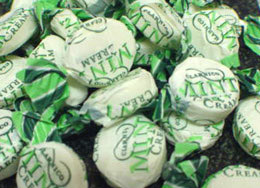This detailed photograph captures a close-up view of a large pile of individually wrapped mints. The image, framed in landscape orientation, showcases a multitude of circular mints, each encased in a predominantly white plastic wrapper. The text "mint ream" is printed in green and black on the wrappers, although it's somewhat hard to read due to the zoomed-in and slightly blurry nature of the photo. The ends of the wrappers are twisted and fan out in various shades of green, adding a splash of color to the overall white background. The mints are jumbled together, forming a dense, overlapping heap. While some of the candies lie sideways or upside down, hints of the surface beneath them are visible between the gaps, particularly toward the lower middle and right. The background, seen in parts of the upper right section of the image, appears to be a marble counter in gray, white, and black, adding a subtle context to the otherwise tightly packed mass of mints.